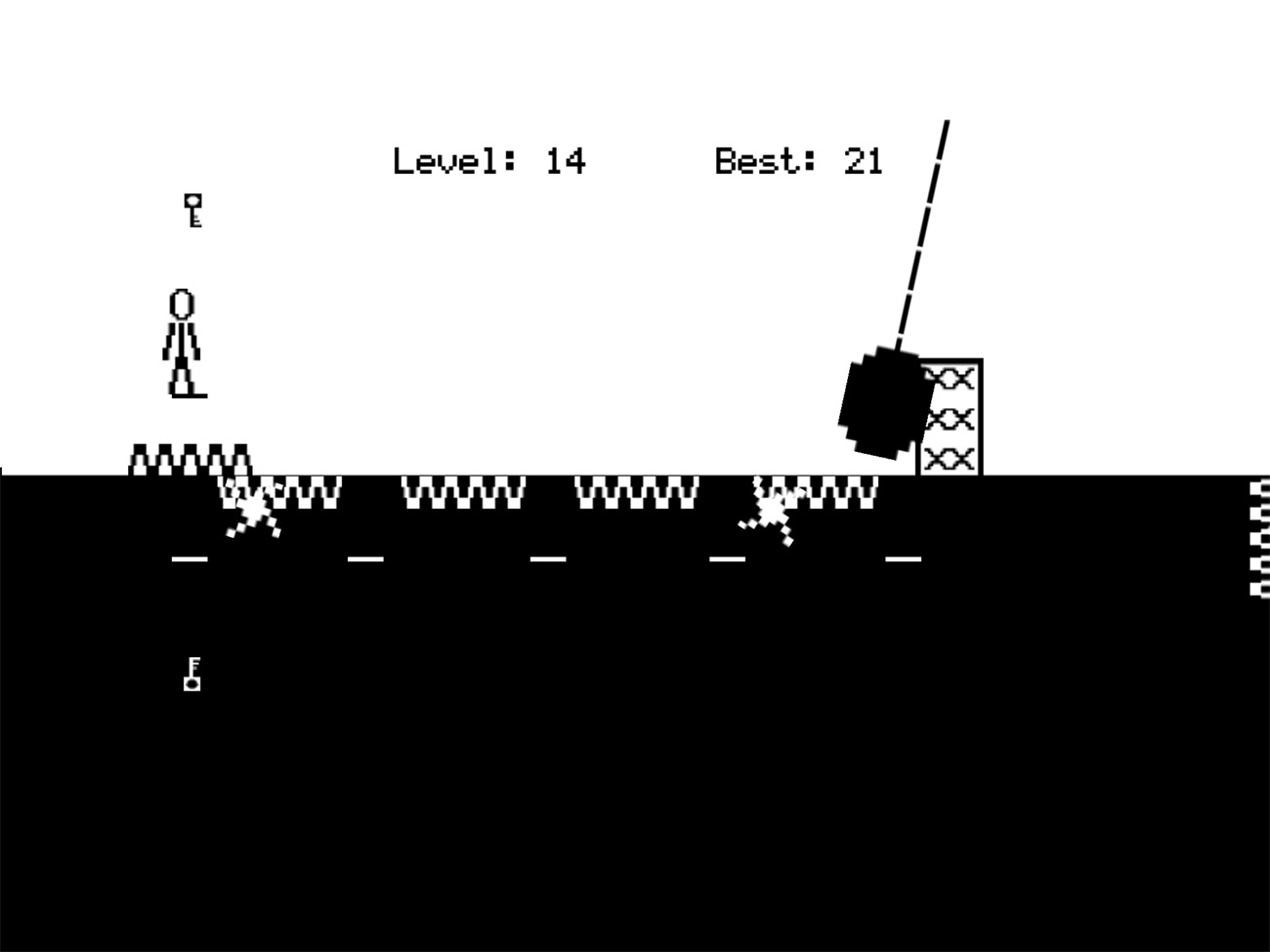The image depicts a screenshot from a very basic, old-style pixelated video game. The screen is divided into two halves: the top half features a white background, while the bottom half is black. Centered at the top of the image, old-school font text reads "level 14, best 21." Directly beneath this text stands a computer-generated stickman, depicted in black pixels. Positioned above the stickman’s head is a small pixelated key.

To the right side of the screen, there's a pixelated wrecking ball attached to a thin line, poised to swing toward a basic, rectangular wall made of pixels, marked with Xs. The bottom half of the image is dominated by a large black rectangle featuring four sets of squiggly white lines at the top, resembling a road, and five white dashes below. Toward the center-left of this black area, another small key is depicted in white pixels.